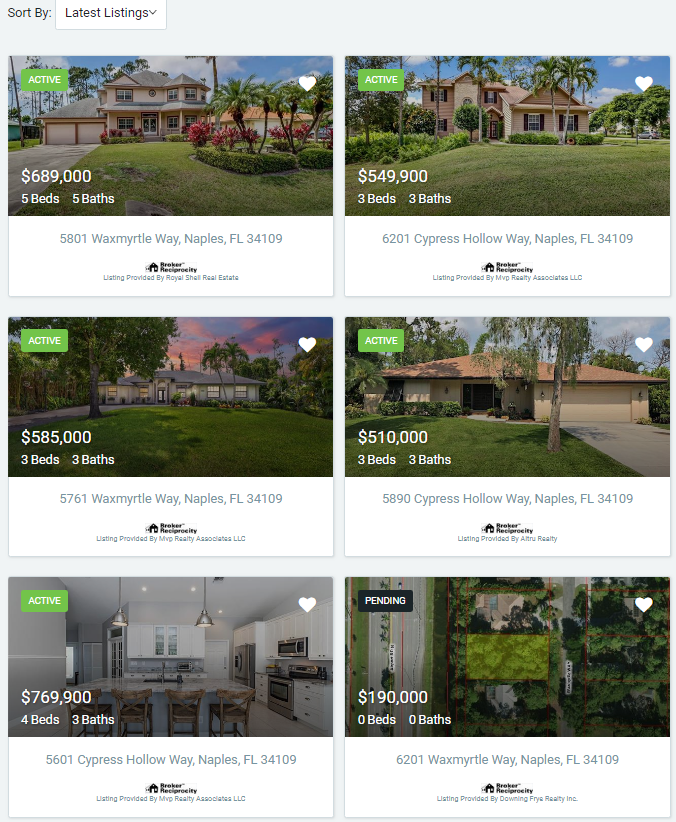Detailed Caption:
The image depicts a real estate website focused on selling homes, characterized by a minimalistic upper banner that does not name the site. The legibility of the text is mostly clear, with a few exceptions. In the upper left-hand corner of the website is a "Sort by" filter, followed by a colon, and then the option "Latest listings" with a drop-down arrow, all presented in white against a light gray banner.

The main body of the site showcases six individual property listings, each with an accompanying photograph. The first image features a spacious house with a large yard, a two-car garage, and an expansive driveway. This property is labeled as "active" and priced at $689,000. It offers five bedrooms and five bathrooms, located at 5801 Wex Myrtle Way, Naples, Florida, 34109.

Adjacent to this is a listing for a home with a substantial lawn adorned with palm trees. This active listing is priced at $549,900 and includes three bedrooms and three bathrooms. 

Beneath these is another active listing displaying a charming house with a visible tree in the yard, priced at $585,000. This property offers three bedrooms and three bathrooms.

The next listing is priced at $510,000 and includes three bedrooms and three bathrooms. 

Following that is a more expensive home listed at $769,900, offering four bedrooms and three bathrooms.

Finally, there is a "pending" listing priced at $190,000 with no specified bedrooms or bathrooms. Each of these properties is neatly displayed for easy browsing by prospective buyers.